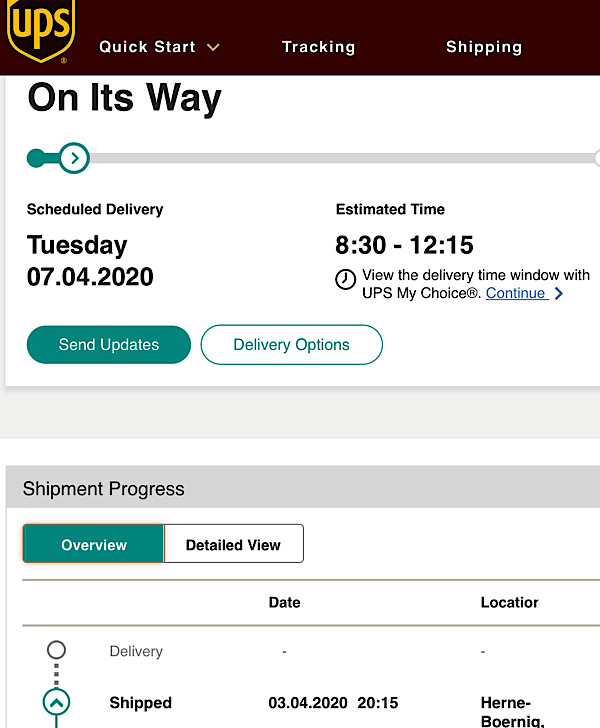In the top left corner is the iconic yellow UPS logo, resembling a badge, with the letters "UPS" prominently displayed in yellow. This logo is set against a dark brown header. To the right of the logo, "Quick Start" is written in small white letters. Below this, an orange downward arrowhead directs attention to the words "Tracking" and "Shipping," both written in white.

The design transitions to a white background, where bold black text announces that the package is "On its way." A long gray line runs horizontally across the image. To the left, there is a green-highlighted section leading into a right-pointing arrowhead within a green-bordered circle. Below this, small black text reads "Scheduled Delivery," which is followed by a larger, bold black font stating the date "Tuesday 07.04.2020."

To the right, smaller black text displays "Estimated Time," and under this, larger bold text—though not as large as the delivery date—shows the timeframe "8:30 - 12:15." Directly below is a clock icon, followed by the message "View the delivery time window with UPS My Choice®," indicating that this feature is registered. The word "Continue" is underlined in blue, suggesting it is clickable, with a blue arrowhead pointing to the right.

At the bottom are two elongated oval icons. The one on the left has a dark green background with the text "Send Updates" in white. The icon to the right features a white background with a green border and the text "Delivery Options" in green.